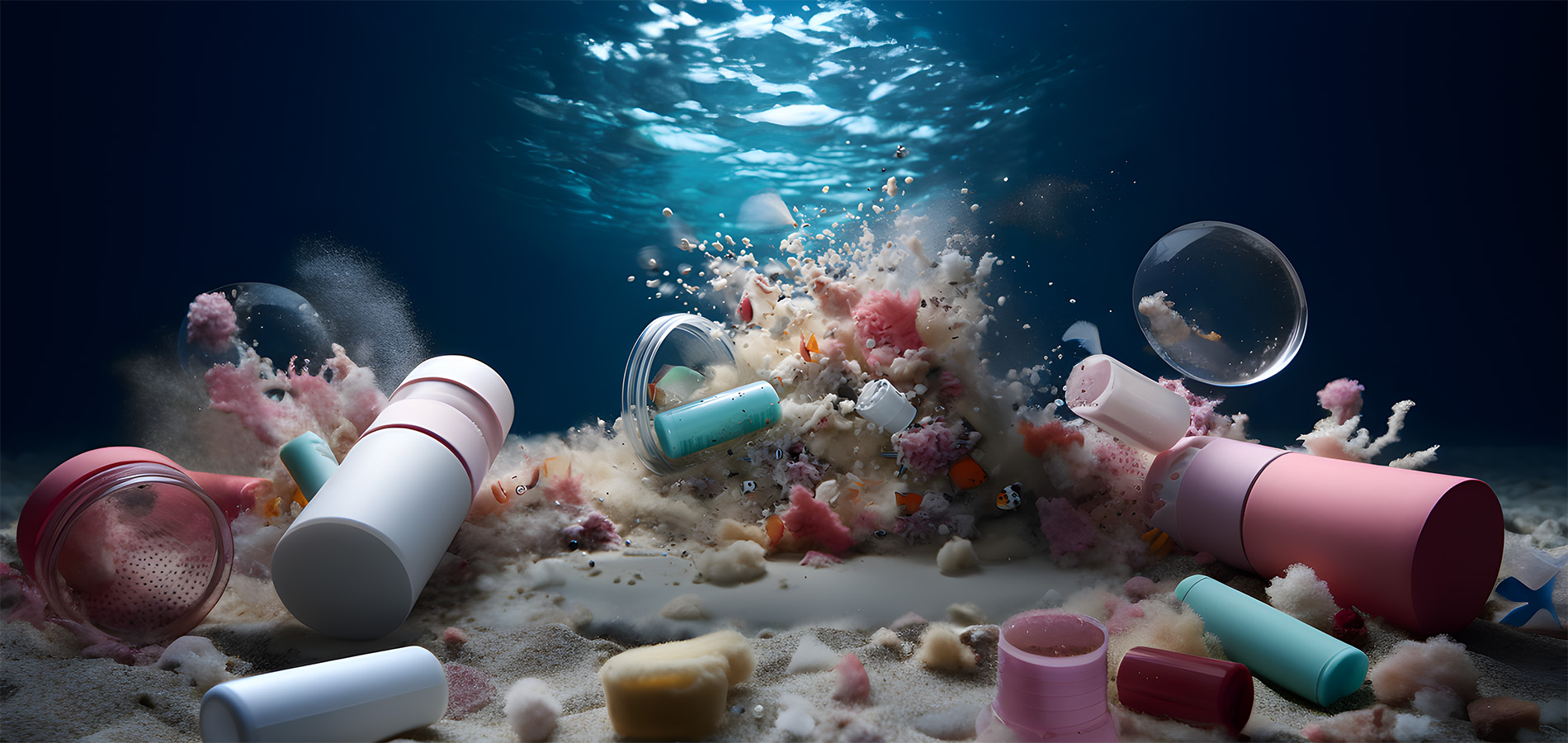The photograph, depicting an underwater scene or possibly a tank, showcases the hauntingly beautiful yet troubling sight of pollution beneath the water. The background is a deep midnight blue, indicating the depths, with a small upper-middle section reflecting aquamarine light, hinting at sunlight permeating the water's surface. Prominently, a large bubble and several smaller ones float in the upper right section, contributing to an eerie stillness.

The sea floor, covered in pale gray sand, is littered with various plastic debris, including tubes and containers in colors such as pink, blue, red, deep maroon, white, and yellow. Some pieces appear to be of broken makeup products, suggesting a range of pollutants. In the mix of plastic refuse, there are also shells scattered among the litter, indicating the adverse effect on marine life. A piece of coral is visible, adding a stark contrast to the surrounding debris and emphasizing the environmental impact. The overall image is a striking visual of underwater pollution, blending natural beauty with the harsh reality of human negligence.